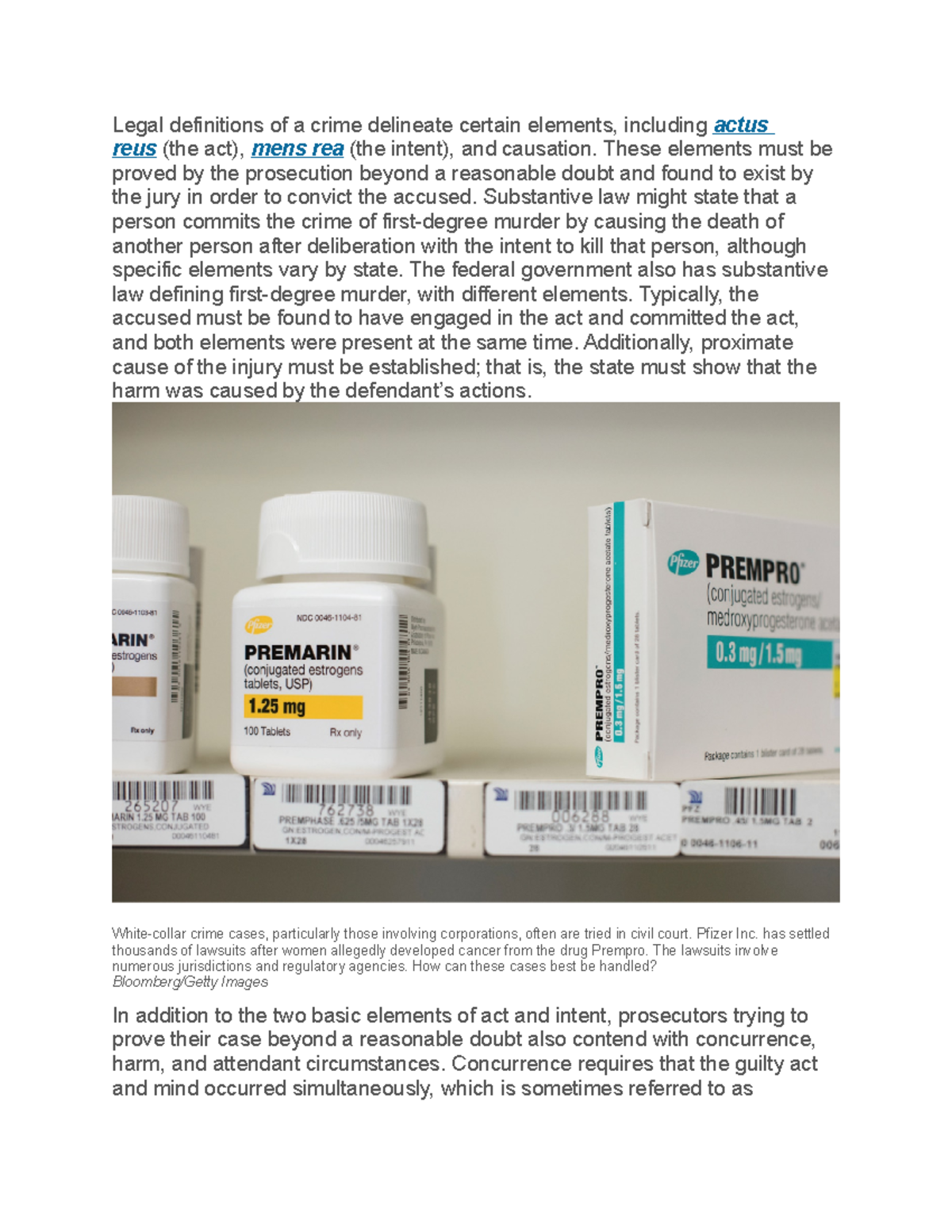Descriptive Caption:

The image displays a screen capture of a medication warning label, featuring extensive textual warnings. Centrally located within the text is a picture depicting three packs of medication neatly arranged on a shelf. The entire image is set against a light gray background. The top segment of the warning label text delves into legal definitions and discusses the elements required to constitute a crime, highlighting terms such as actus reus (the act), mens rea (the intent), and causation. It explains that these elements must be demonstrated by the prosecution beyond a reasonable doubt for a jury to convict the accused. Furthermore, it elaborates on the crime of first-degree murder, detailing its requirement for causing the death of another person with premeditated intent to kill, while noting that the specific legal elements may differ by state.